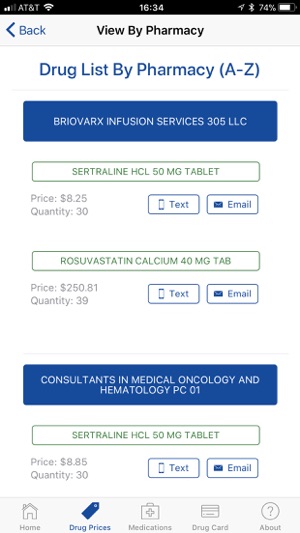The webpage displays various elements organized into different sections, each featuring drug information and options for contacting pharmacies. 

At the top, a navigation bar contains a back button alongside the word "Back" in blue. A nearby option labeled "View by Pharmacy" is in black within a gray rectangle.

Below this, a blue header reads "Drug List by Pharmacy A through Z." The first entry under this header is "Bryo Barks Infusion Services 305 LLC" written in white text within a blue rectangle.

Under a gray-outlined rectangle, the first drug listed is "Sertraline HCL 50 mg tablet" with details: price of $8.25 for a quantity of 30, positioned to the left. To the right are options for "Text" and "Email" communications.

Following that, in another gray-outlined section, "Rosuvastatin Calcium 40 mg tab" is listed with a price of $250.81 for a quantity of 39, again on the left. Next to it, the right side offers "Text" and "Email" options, the "Text" button within a blue outline.

A blue rectangle with white text reads "Consultants in Medical Oncology and Hematology PCO 1," followed by another entry for "Sertraline HCL 50 mg tablet" priced at $8.85 for a quantity of 30 on the left, with "Text" and "Email" options on the right.

At the bottom of the page, a gray rectangle displays icons for Home, Drug Prices, Medications, Drug Card, and About sections, providing easy navigation to these areas.